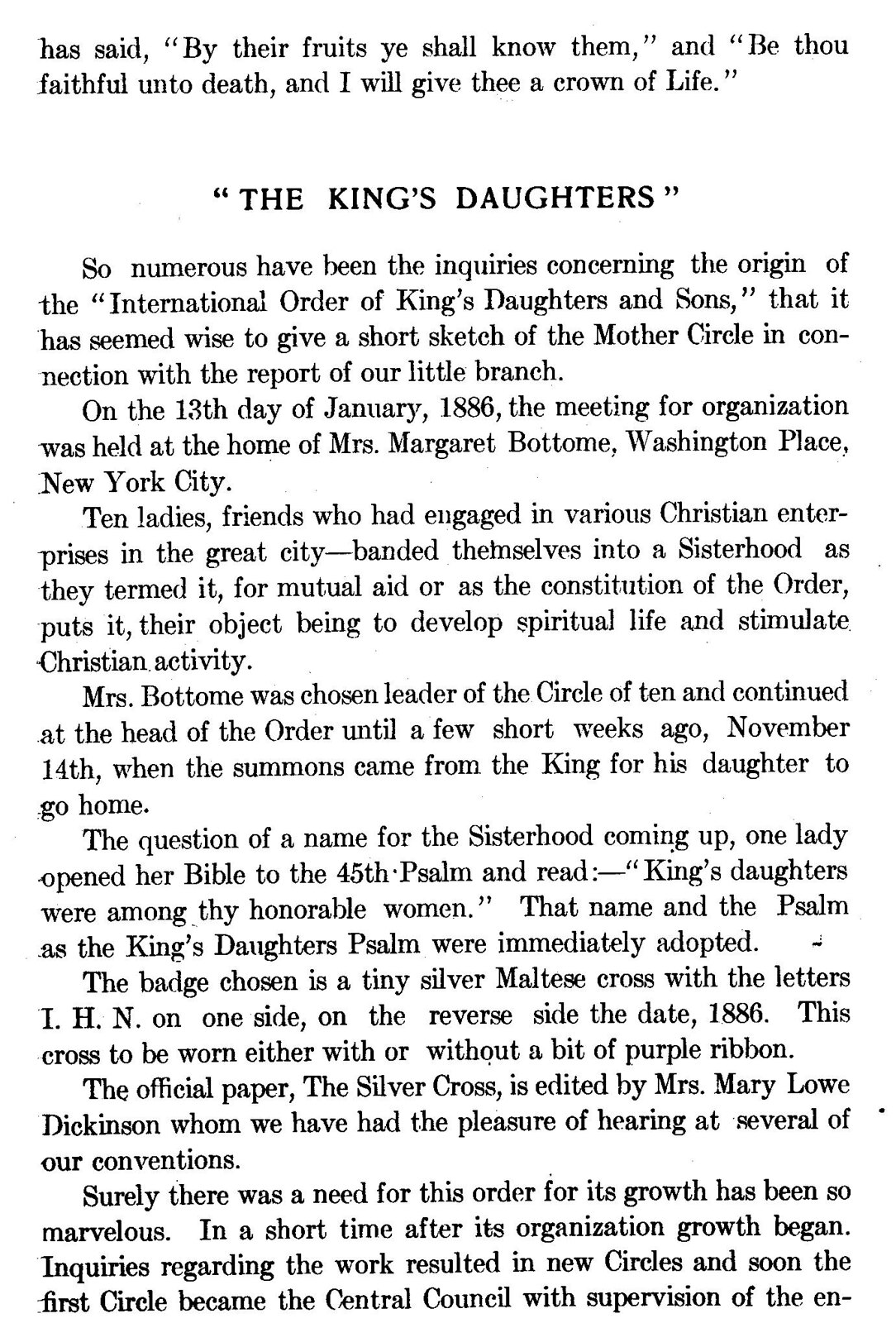This is a page on a white background with extensive text. The page begins with a partially cut-off inscription, "By their fruits ye shall know them, and be thou faithful unto death, and I will give thee a crown of life." Below this, in uppercase black print and parentheses, is the title "The King's Daughters." The text starts by addressing numerous inquiries about the origin of the International Order of King's Daughters and Sons, and therefore provides a short sketch of the Mother's Circle alongside a report of a smaller branch.

The narrative recounts that on January 13, 1886, an organizational meeting took place at Mrs. Margaret Bottom's home at Washington Place, New York City. At this gathering, ten ladies who were friends and had engaged in various Christian enterprises in New York City formed a sisterhood for mutual aid. The Constitution of the Order states that their purpose was to develop spiritual life and stimulate Christian activity.

Mrs. Bottom was elected as the leader of this Circle of Ten and served as the head of the order until recently, November 14, when she passed away. The group faced the question of a name for the sisterhood; one lady opened the Bible to the 45th Psalm and read, "King's daughters were among the honorable women," leading to the immediate adoption of the name "The King's Daughters."

The badge chosen for the sisterhood is a small silver Maltese cross, with the letters IHN on one side and the date 1886 on the reverse. This cross could be worn with or without a bit of purple ribbon. The official paper of the order, titled "The Silver Cross," is edited by Mrs. Mary Lowe Dickinson, who has spoken at several of their conventions. The text culminates by emphasizing the rapid growth and widespread inquiries about the order, resulting in the formation of new circles, and establishing the first circle as the Central Council overseeing the movement. The text cuts off, not completing the final sentence.